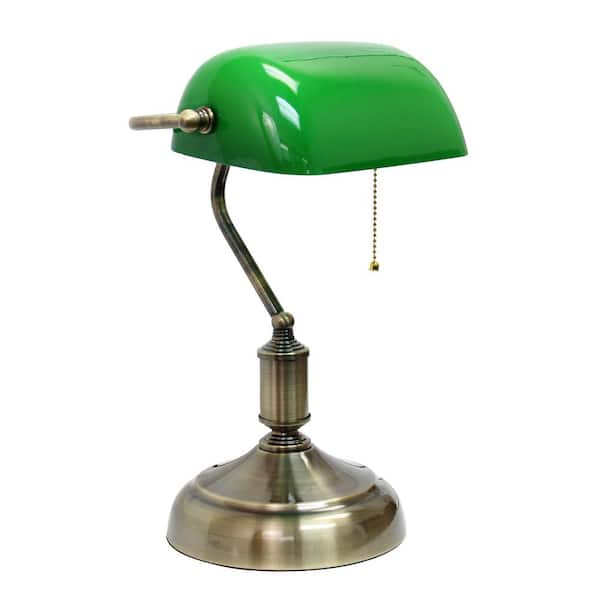The image features a vintage-style desk lamp set against a plain white background. The lamp has a circular metal base, likely brass or a similar reflective material. Extending upwards from the base is a rod, which may be adjustable and appears to be attached to a hinge, allowing for vertical rotation. The lamp's neck curves elegantly, culminating in a green translucent glass shade that resembles a scoop. A small metal handle is visible on the side of the shade, possibly for adjusting its angle. A beaded pull chain hangs from the top of the lamp, used to turn it on or off. The overall design suggests the lamp could date back to the 1940s, exuding an old-time charm with its classic and attractive aesthetic.